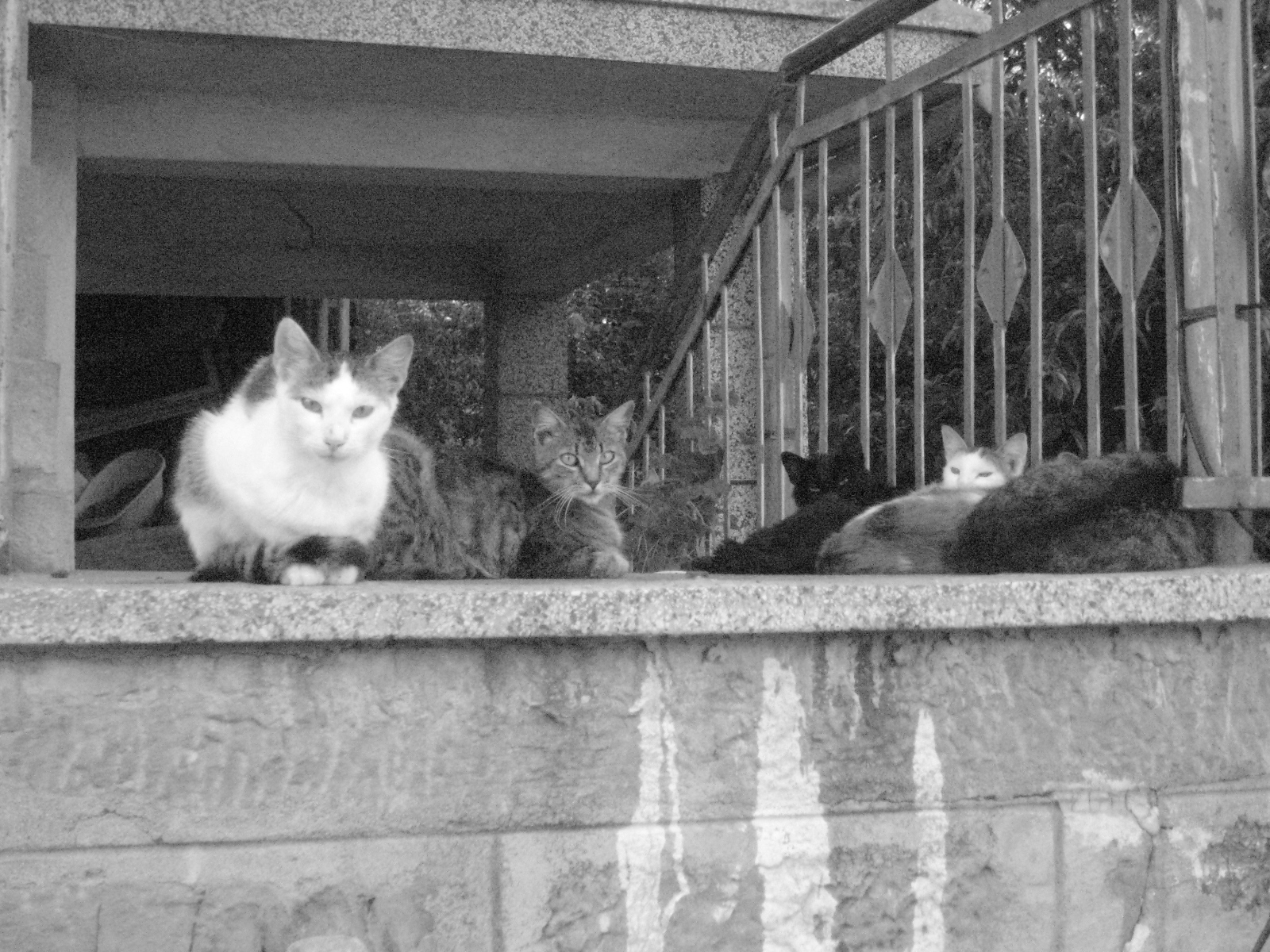The image captures five cats lounging atop a stone wall with a slightly wider concrete ledge at the top, situated near a railing by a multi-story apartment building. Four of the cats are facing the camera, while the fifth cat, closest to the viewer and curled up, has its head hidden. Among the feline group, two are gray, one is black, and the others are multi-colored, with combinations of gray, white, brown, and black fur. The wall is adjacent to a staircase with a railing that seems to ascend from the ground to meet the wall under a wooden structure resembling a landing porch. The setting appears to be slightly below street level, suggesting a lower apartment floor. The cats are in various relaxed poses, creating a peaceful and cozy scene.